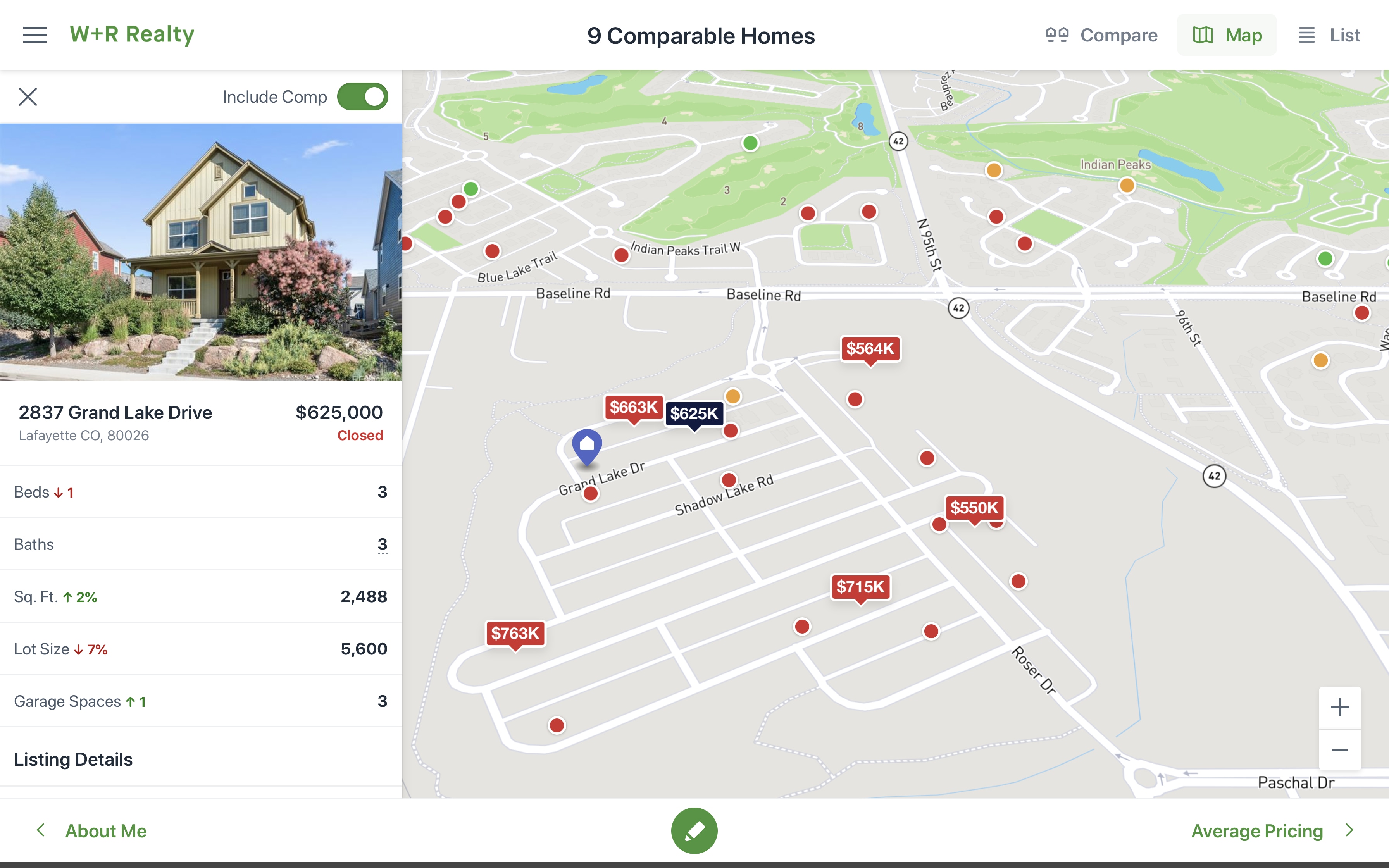The image depicts a user interface, likely intended for either a tablet application in landscape mode or a responsive website. The layout is quite organized and visually balanced. 

The header section stretches across the top, starting with three horizontal lines (indicative of a menu icon) on the upper left. Following this, the text "W+R Realty" is prominently displayed. Further to the right, the phrase "Nine Comparable Homes" is positioned, providing users with context for the listings. Additionally, there are icons labeled "Compare" and "Map," which are positioned next to the phrase. The section concludes with an icon featuring four horizontal lines (possibly another menu-related function) and a "List" label.

The body of the webpage is divided into two main columns. On the left column, the selected house's detailed information is presented. This includes the address, city, state, zip code, price, and various specific features of the house. To the right, a map offers a visual representation of different listings, showing their locations along different streets along with the corresponding prices.

At the bottom, the footer is systematically arranged. On the lower left, there is a left arrow icon labeled "About Me." Centrally, there's a distinctive white pencil logo in a green circle, suggesting an editable feature or note function. Finally, on the lower right side, there is an "Average Price" label with a right arrow icon, potentially leading to additional price data.

This detailed arrangement ensures users can efficiently navigate and compare real estate listings visually and textually.